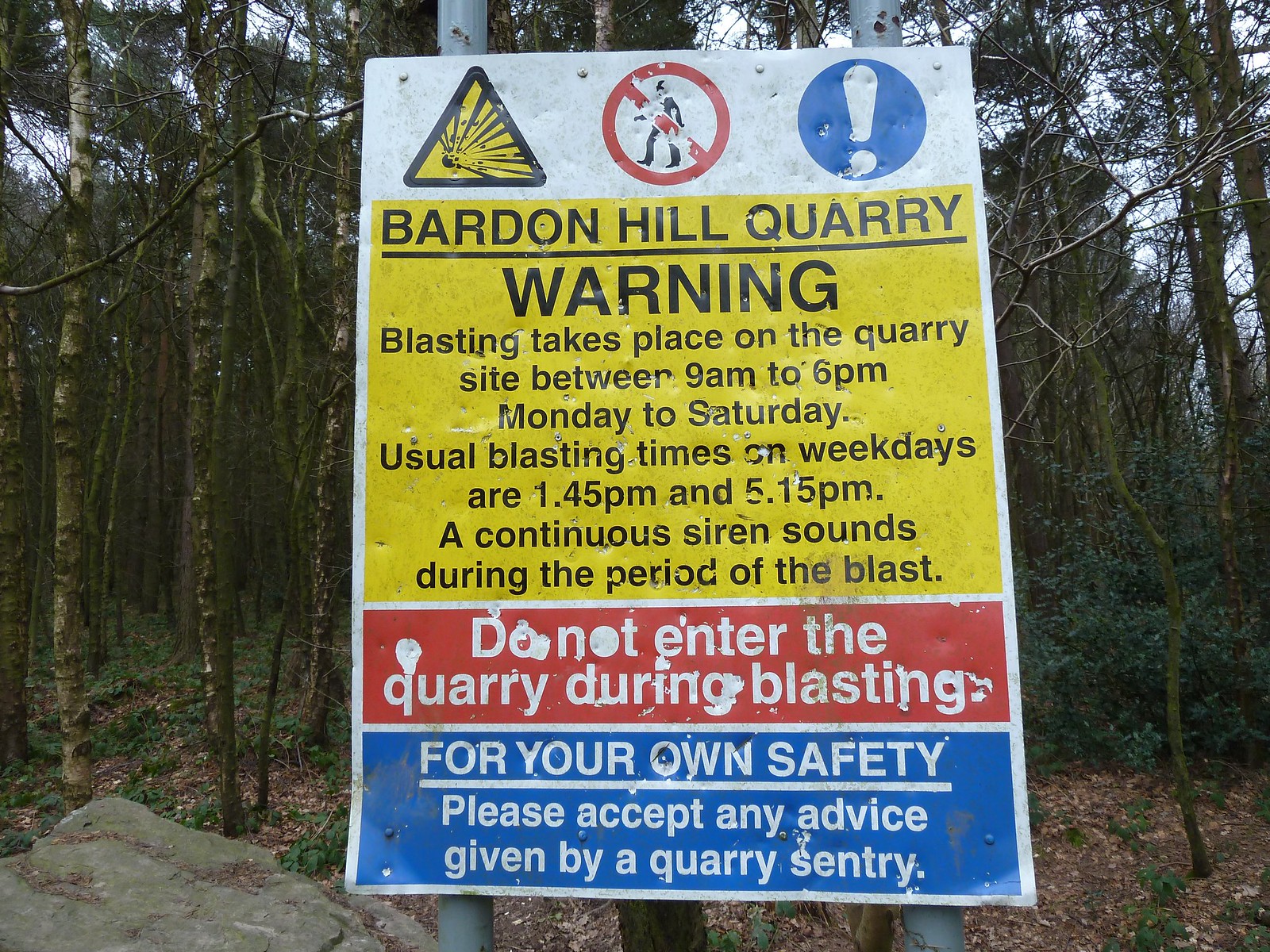The photograph depicts an outdoor setting with a dense backdrop of trees and leaves scattered on the ground, accompanied by a noticeable rock in the bottom left corner. Prominently positioned in the center is a weathered metal sign, affixed to two metal posts anchored into the ground. The sign states: "Barden Hill Quarry Warning. Blasting takes place on the quarry site between 9 a.m. to 6 p.m. Monday to Saturday. Usual blasting times on weekdays are 1:45 p.m. and 5:15 p.m. A continuous siren sounds during the period of the blast. Do not enter the quarry during blasting. For your own safety, please accept any advice given by a quarry sentry." At the top of the sign, there are three distinct safety symbols: a yellow caution triangle representing blasting, a no-entry symbol featuring a crossed-out person, and a blue circle with a white exclamation mark. The scene is bright and clear, indicating that the photo was taken during the daytime, with ample natural light highlighting the sign and its details against the lush, green environment.